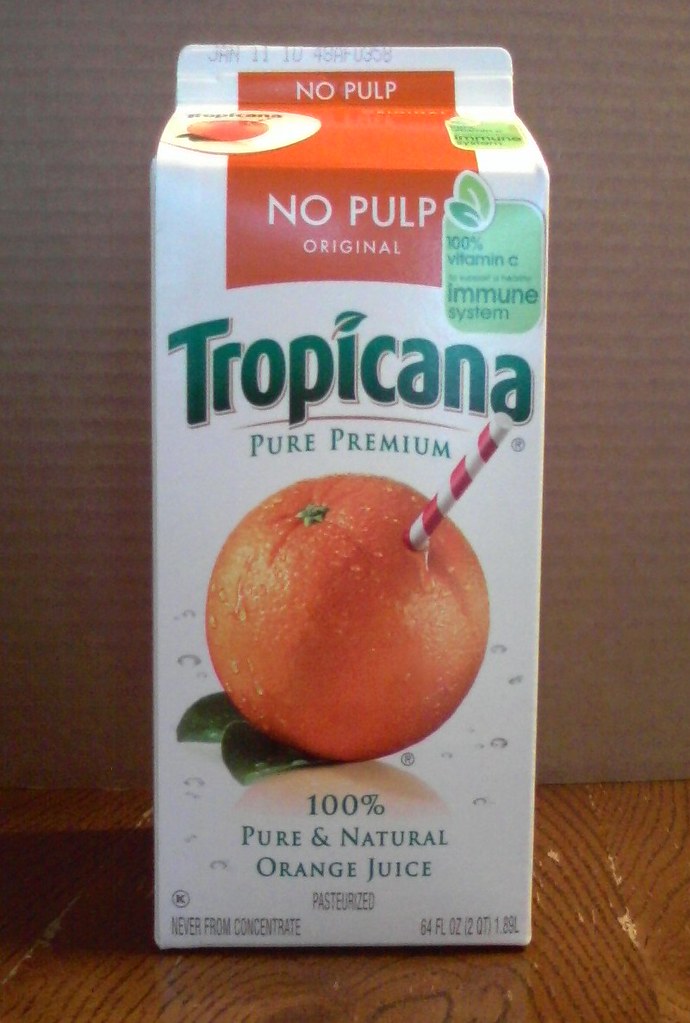This image features a carton of Tropicana orange juice placed on a brown table adorned with intricate black lines. The carton has a predominantly white background with an orange top where the words "No Pulp" are clearly stated in white text. Just beneath the top, there is a white circular logo accompanied by an orange graphic on the left and a green logo to the right.

Midway down the carton, against an orange backdrop, "No Pulp" and "Original" are again highlighted in white text. To the right, a mint green label accentuates the carton, proudly claiming "100% Vitamin C" and "Immune System Support" in green text. Below this, the brand name "Tropicana" is prominently displayed in green, with the letter "i" creatively dotted by a leaf. The phrase "Pure Premium" follows, also in green.

A striking image of an orange with a red and white striped straw is located towards the lower right, reinforcing the product's freshness. The bottom of the carton is stamped with the information "100% Pure and Natural Orange Juice" in green text, completing the detailed visual description.